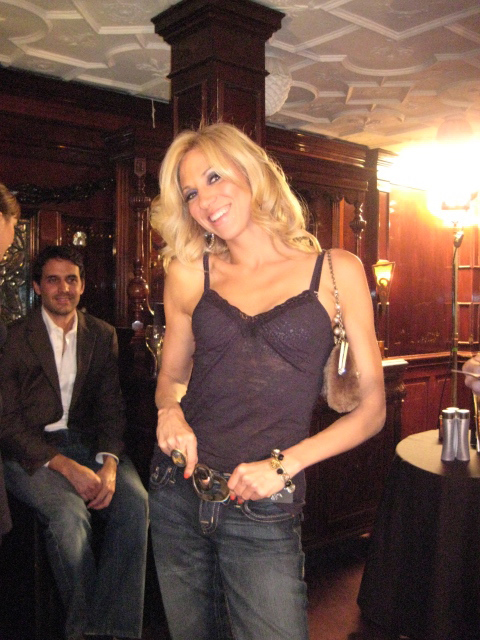The image captures an indoor setting that appears to be a bar or a basement, featuring a central figure—a woman with long, wavy blonde hair—smiling directly at the camera. She is wearing a purple tank top with thin straps, denim jeans, and has a small, fluffy purse slung over her right shoulder. Her muscular shoulders are noticeable, and she's wearing bluish eye shadow. The environment includes a white ceiling with designs, brown furniture, and a prominent brown beam reaching up to the ceiling. Surrounding her are cabinets, counters, and black tables with various items on them. In the background to the left, a man dressed in jeans and a brown suit jacket sits on a bar stool, also smiling. The color palette includes yellow, brown, orange, tan, black, blue, and brown, highlighting the cozy and warmly lit atmosphere of the space.